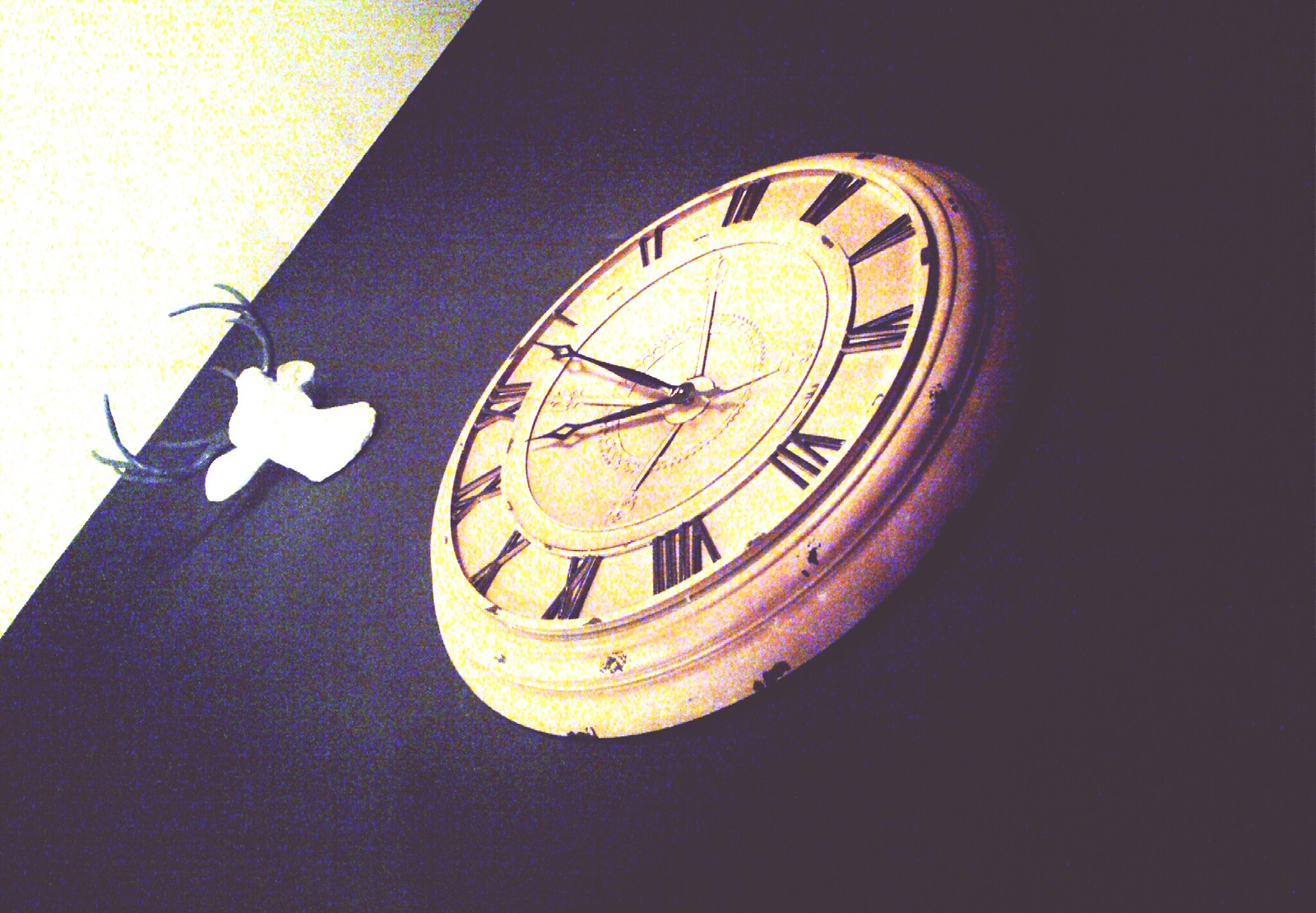This image captures a unique perspective from floor level, looking up a black-walled room towards a white ceiling. Dominating the scene is a large, antique off-white analog clock with black Roman numerals and metal hands, set at approximately 11 o'clock. The clock is positioned at a slant, so the number two faces upwards rather than the number twelve, highlighting the side view. Adjacent to the clock is a stark white deer head with black antlers. The deer head is nearly featureless due to overexposure, giving it a ghostly appearance. The photo is filtered in such a way that the right side is darkened, the center is lightened, and the left side is also in shadow, creating a striking visual effect.